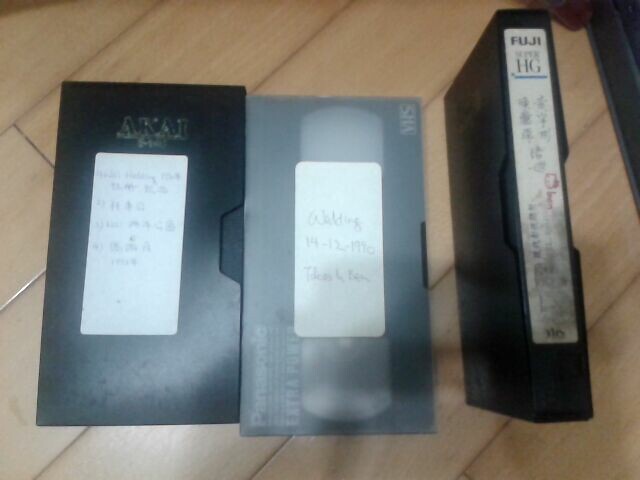The photograph is an overhead shot of three vintage VHS cassette tapes arranged side by side on a light oak wooden table or floor. The VHS cassette on the far left is outside of its black dust jacket, displaying a white sticker with the handwritten label "Wedding, 14-12-1990," indicating it might be a homemade recording. The middle cassette is flat and has a gray section with possibly faint writing; it might have Panasonic branding in the lower corner and a clear area in the center. The third VHS cassette, on the right, is inside its black dust jacket and stands vertically. This cassette features a white label that reads "Fuji HG," followed by Japanese characters. Each cassette and its cover is black, and the overall image is somewhat out of focus, but the wooden background with its oak patterns is distinguishable.